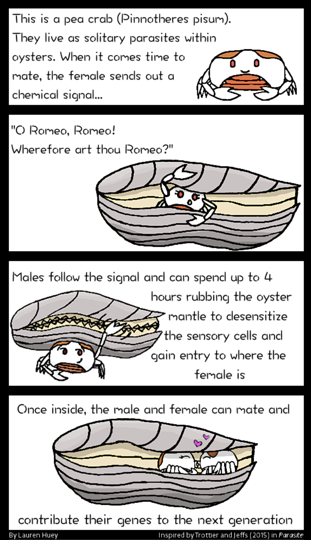The image is a detailed illustration about a peat crab, scientifically known as Pinotheris pisum, designed in a vertical rectangular format with a black border. The rectangle is divided into four panels, each containing black text and colored drawings. 

**First Panel:** At the top, it introduces the crab with the text, "This is a pea crab," followed by its scientific name in parentheses. Beneath the initial line, four lines of text describe the crab’s characteristics and behavior. To the right of this text, there is an illustration of a peat crab colored in white and brown, showcasing its prominent claws and a gray shell-like structure.

**Second Panel:** This section has two lines of text accompanied by an illustration to the right, which continues to describe the crab's parasitic nature and its relationship with oysters.

**Third Panel:** This part features an image at the bottom left and five lines of text to the right, connected by a black line at the top. The text explains the female crab’s mating signal and the male's response, detailing the desensitization of the oyster's sensory cells to gain entry.

**Fourth Panel:** The final section has a text line at the top and another at the bottom, flanking an illustration in the center. This part depicts the mating process and the genetic contribution to the next generation. Tiny, unreadable white text is positioned within the black border on the left and right edges.

The overall setup and style blend text with illustrations to narrate a short, informative story about the life and mating behaviors of the pea crab.